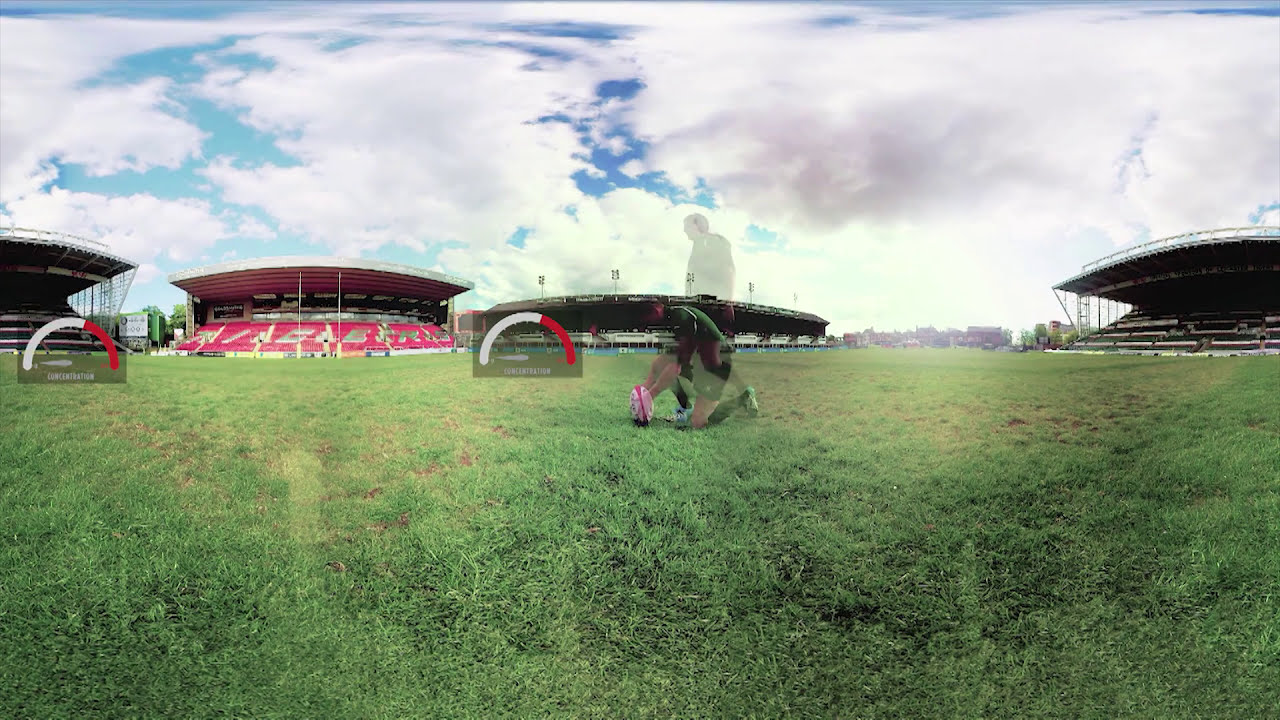The photograph captures a vivid outdoor sporting scene under a partly cloudy sky. A bright blue background is highlighted by numerous puffy white clouds, some having grayish bottoms, and sunlight peeking through on the right side. Below this, a sprawling green grass field dominates the lower portion of the image, signifying an athletic stadium.

In the foreground, a man dressed in a green uniform is kneeling on the grass, placing a football in front of him; the football appears to have white and red stripes. This central activity is framed by various stadium structures. On the right side, a covered seating area with an open front and sides is visible, featuring metal roofing. The middle background showcases additional bleachers accented with multiple stadium lights, also with an open design. On the left side, another set of bleachers stands out with red seating, framed by a metal and white roof, also open on the front and sides.

Interestingly, the stands seem to have letters that aren’t decipherable and possibly not in English. Some imposed, shadowy figures and semicircular shapes in the image further add a layered depth, though these elements don't appear to be part of the physical environment. Overall, this detailed scene captures the serene yet dynamic atmosphere of a football stadium.